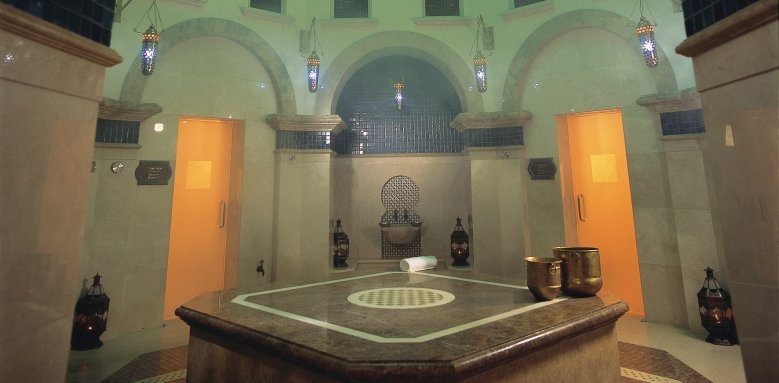This photograph captures the intricate design of an indoor hall that resembles either a grand church or a bathhouse with Middle Eastern design elements. The focal point of the image is a large square table in the foreground, made of alternating dark and light granite. On this table are two ornate silver urns and a circular centerpiece with greenish or grey elements. This table is encircled by additional vases and what look like white rolls of cloth.

The background features three towering arches supported by two columns, which frame an opening that leads to a sanctuary or altar area. Within this middle arch, a stand with curved elements and statues is flanked by two large vases. The walls are adorned with sculpted arches and marble, lending a shiny, reflective quality to the entire scene. 

Above the arches, elaborate sconces or lanterns hang suspended from the ceiling, providing illumination. On either side of the arches, there are wooden doors with black handles that appear to emit a warm, orange glow, suggesting that the interior is well-lit. The marble flooring adds to the elegance of the space. This intricate and opulent setting, complete with its shimmering surfaces and detailed decor, captures the ambiance of a sacred or ceremonial space.